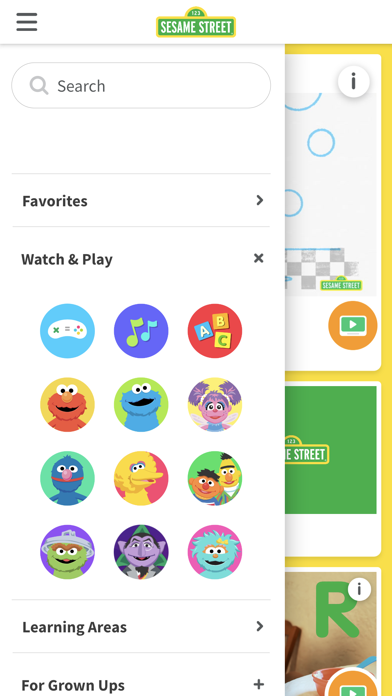Screenshot of the Sesame Street app on a smartphone. The interface features a hamburger menu in the upper left corner, with the iconic Sesame Street logo positioned at the top, displaying "1, 2, 3" on a green street sign with white text and a yellow border. The main content area offers various background options and images, including elements related to counting or the letter "R," which are partially obscured by a slide-out menu on the left. This slide-out menu features a drop shadow, indicating it is layered above the rest of the interface.

At the top of the slide-out menu, there is a search field, followed by options for "Favorites" and "Watch and Play." The "Watch and Play" section displays 12 icons arranged in a 3x4 grid. These icons represent different interactive elements such as a game controller, music notes, alphabet blocks, and characters including Ernie, Cookie Monster, a little girl, Grover, Big Bird, Ernie and Bert together, Oscar the Grouch, The Count, and an unidentified blue character.

Below this section is a label titled "Learning Areas," followed by a button labeled "For Grown Ups" accompanied by a plus sign. The overall layout is simple and white, designed to be user-friendly for children, while also providing options for adults to access control settings.